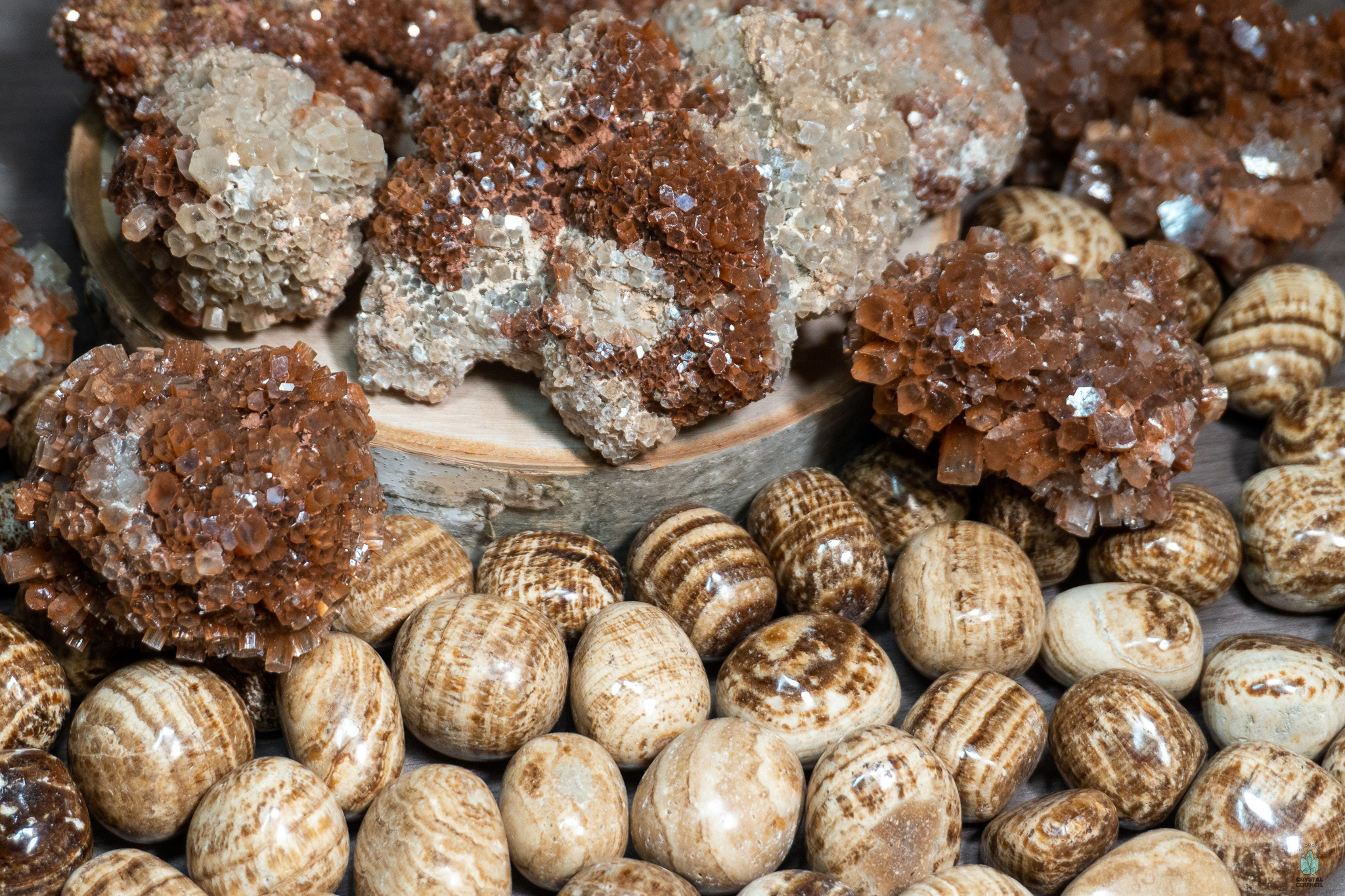The image features an organized arrangement of geological specimens, prominently showcasing a combination of polished and crystallized rocks. Central to the scene are several polished stones with distinctive brown and white stripes, resembling large, smooth eggs. These stones are primarily located in the bottom third of the image, scattered across what appears to be a flat surface or table. Surrounding these polished stones are numerous geode-like rocks, notable for their rough, crystalline formations that glint in the light. Predominantly featuring hues of tan, dark brown, and off-white, these geodes display a spectrum of sparkling crystal interiors that capture the viewer's attention.

In the middle left section of the image, set against a wooden stump, is a large rock with embedded quartz crystals, which extends to the top left corner, further showcasing its intricate crystalline structure. The top right area contains additional quartz-laden rocks, their impressive formations glistening with a mix of white and brown crystals. These crystalline rocks dominate the upper portions, adding texture and a sense of depth to the scene. The overall composition suggests a curated display, potentially for a website dedicated to geology enthusiasts or rock collectors, highlighting the intricate beauty and variety of natural mineral formations.